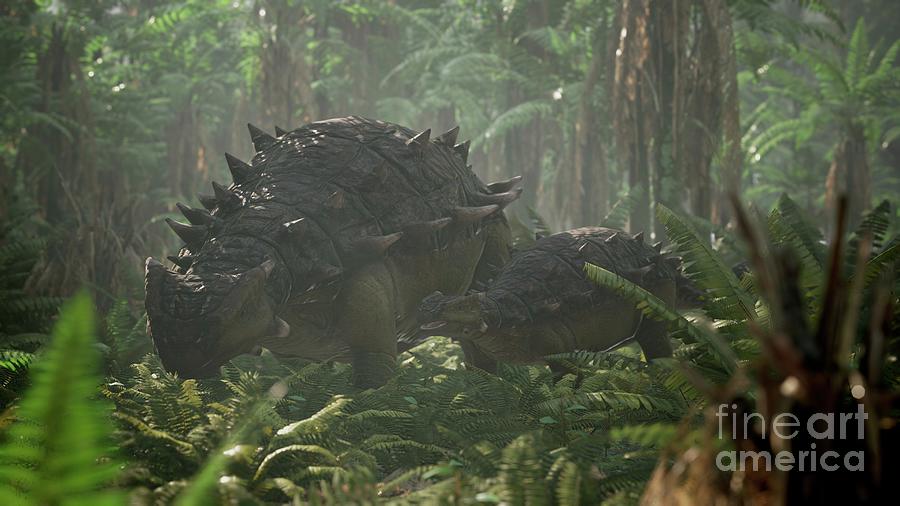This image, adorned with a watermark from Fine Art America in the bottom right corner, depicts a CGI-rendered scene featuring two dinosaurs, likely Stegosauruses, in a lush, verdant jungle setting. The dinosaurs are depicted in a lifelike yet clearly animated style, walking on all fours with distinctive flat heads, rounded backs, and prominent spikes protruding from their backs, giving them a somewhat turtle-like appearance. They are situated in a dense forest environment replete with towering trees, including at least one massive tree, and a profusion of green vegetation that extends into the foreground. The ground is densely covered with shrubs and smaller plants, some of which are blurred in the immediate foreground, emphasizing the depth of the image. The overall scene is one of rich, dense foliage typical of a tropical rainforest, encapsulating the dinosaurs in their natural, prehistoric habitat.